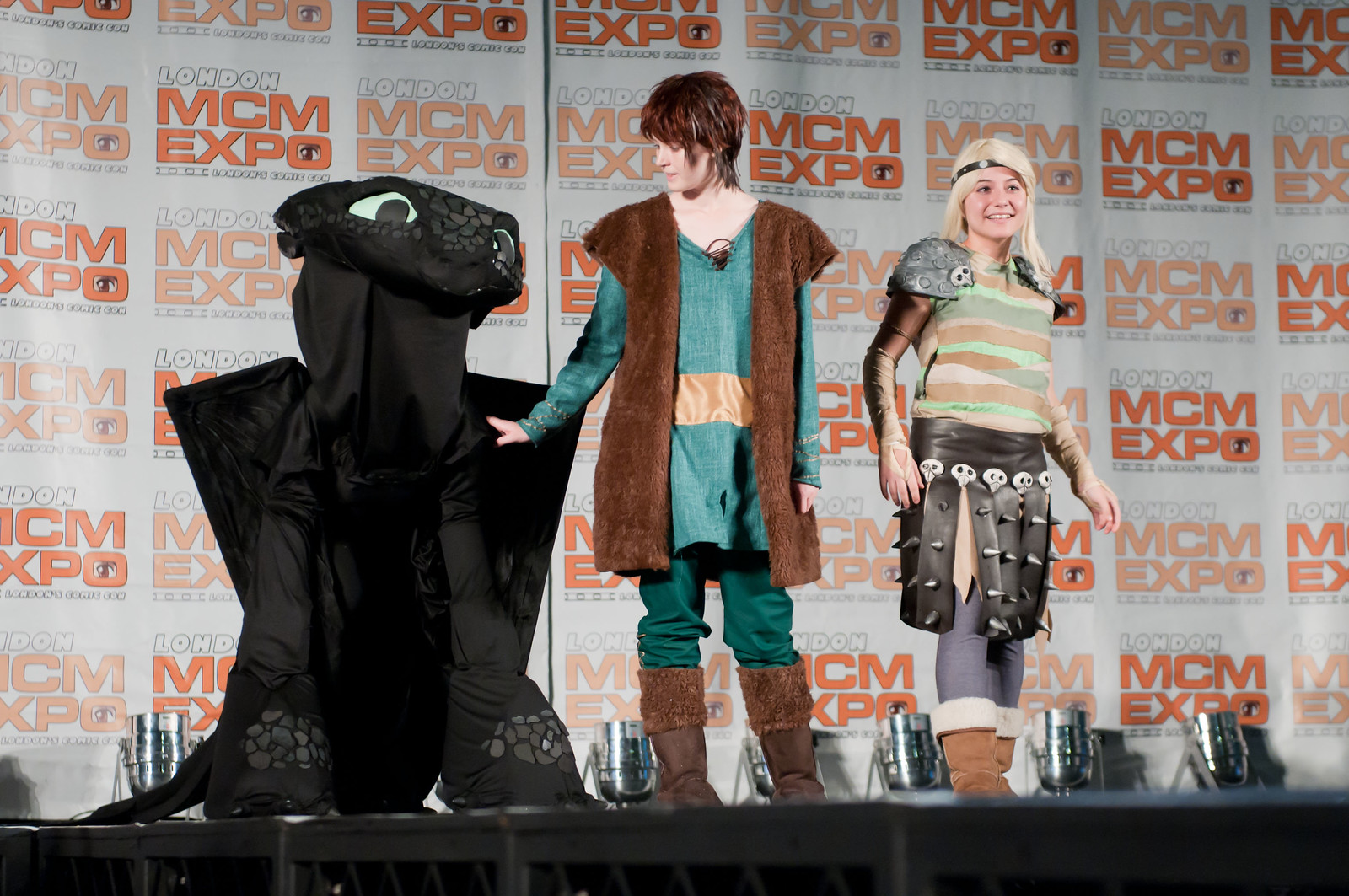This photograph captures a vibrant scene at the London MCM Expo, where three young cosplayers are showcased on stage against a backdrop emblazoned with "London MCM Expo" in bold white letters outlined in black with red "MCM Expo" beneath. The trio embodies characters from "How to Train Your Dragon" with impressive detail. 

On the far left, an individual is entirely encased in an intricate black Toothless costume, complete with large eyes, short triangular wings, and a cloth-like texture, reminiscent of a mascot suit. Center stage stands a young man clad in a historically inspired green tunic with brown boots and a long brown vest, strikingly similar to a Middle Ages or Star Wars aesthetic. His attire includes turquoise pants, adding a modern twist. He rests a hand on Toothless' shoulder while gazing with affection.

To his right is a young woman portraying a fierce warrior akin to Xena, the warrior princess. She sports a striped tunic with shades of light orange and turquoise, along with striking pauldrons, a leather skirt adorned with metal spikes, grayish leggings, and sturdy brown boots. Her blonde hair is held back by a dark headband, emphasizing her character's boldness. The woman smiles warmly, adding to the scene's dynamic and engaging atmosphere, complemented by the spotlight illuminating the cosplayers.